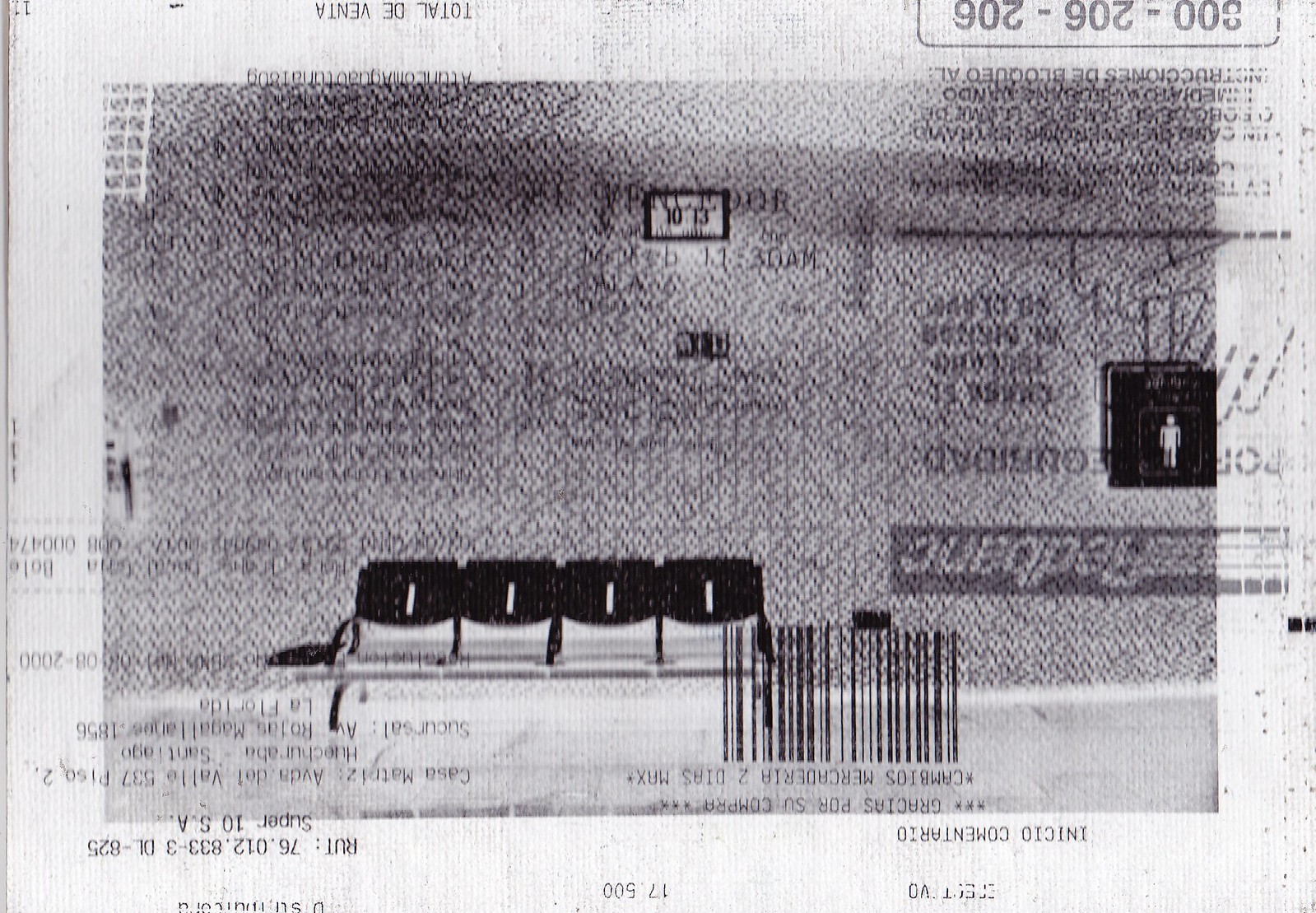This black and white image features what appears to be a ticket, potentially for seating arrangements. The image is viewed from an unusual angle, rendering the text and numbers upside down and reversed. In the foreground, four black seats are clearly visible. A barcode is located in the lower right-hand portion of the image, adjacent to these seats.

In the right-hand corner, the numeric sequence "300-206-206" is prominently displayed. On the upper left-hand side, amid upside-down and reversed text, the phrase "TOTAL DA VENTA" is discernible, suggesting the ticket might be in a different language.

Additionally, there is a black tunnel-like mark featuring a white symbol of a person in its center. The lower half of the image contains most of the key information, including the barcode and the seating. A potential date and time can be observed in the left-hand corner, although it is somewhat obscured by the perspective.